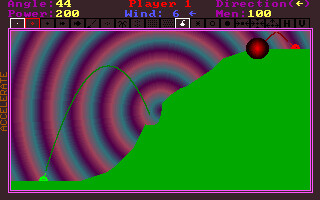The image depicts a small game screen, likely from a phone or tablet. At the top, various game statistics are displayed in bright colors on a purplish-gray background, including "angle" in purple, "44," "power" at "200," "player 1" in red, "wind" at "6" in blue, and "direction" with an arrow pointing left alongside "M-E-N 100" in purple. The main focus of the image is an uneven green hill that starts from the bottom left corner and ascends diagonally to the top right corner, where a small red light or a red and black circle is located. A small green character, about a fourth of an inch tall, is at the bottom left, shooting a curved green line upwards. The background features a colorful bullseye pattern with concentric circles in shades of blue, purple, and pink.